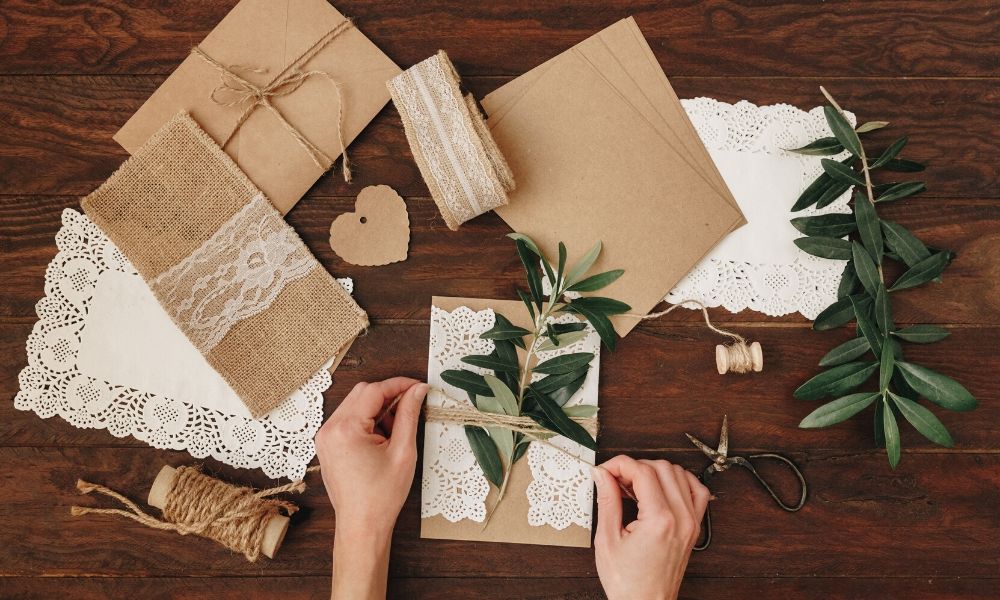In the image, two hands are meticulously crafting greeting cards on a dark-stained slatted wooden tabletop. The craft utilizes natural brown paper, akin to grocery bag material, which has been shaped into envelopes and decorated with delicate white lace and sprigs of greenery. Hearts cut out of the same brown paper add to the rustic charm. The hands are seen tying natural-colored twine around the envelopes, some of which are layered with paper doilies and burlap ribbons. The tabletop includes various elements of this creative process: an aged, rusty pair of scissors, a loose roll of lace, additional stems and branches, and a roll of string. The overall scene evokes a sense of handcrafted elegance, blending natural textures with vintage-inspired details.